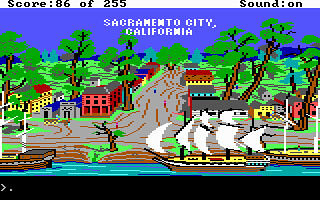In the video game image, the top left corner displays a score of 186 out of 255, while the top right indicates that the sound is active. The bottom of the screen features a black command bar. The scene is set around a blue river, which features dark blue, light blue, and black lines running through it. There are two ships on the river: one on the left and another on the right. The ship on the right has multiple white sails, a yellow top, and a brown hull with yellow and white accents. Surrounding the river are multiple gray roads extending in various directions. The buildings in the scene include a red structure on the left with a gray chimney and a gray rooftop, and a white building on the right with a gray rooftop. The environment is lush with trees featuring different shades of green leaves. The sky is a clear blue, and the text "Second worst city in California" is displayed prominently at the top of the image.